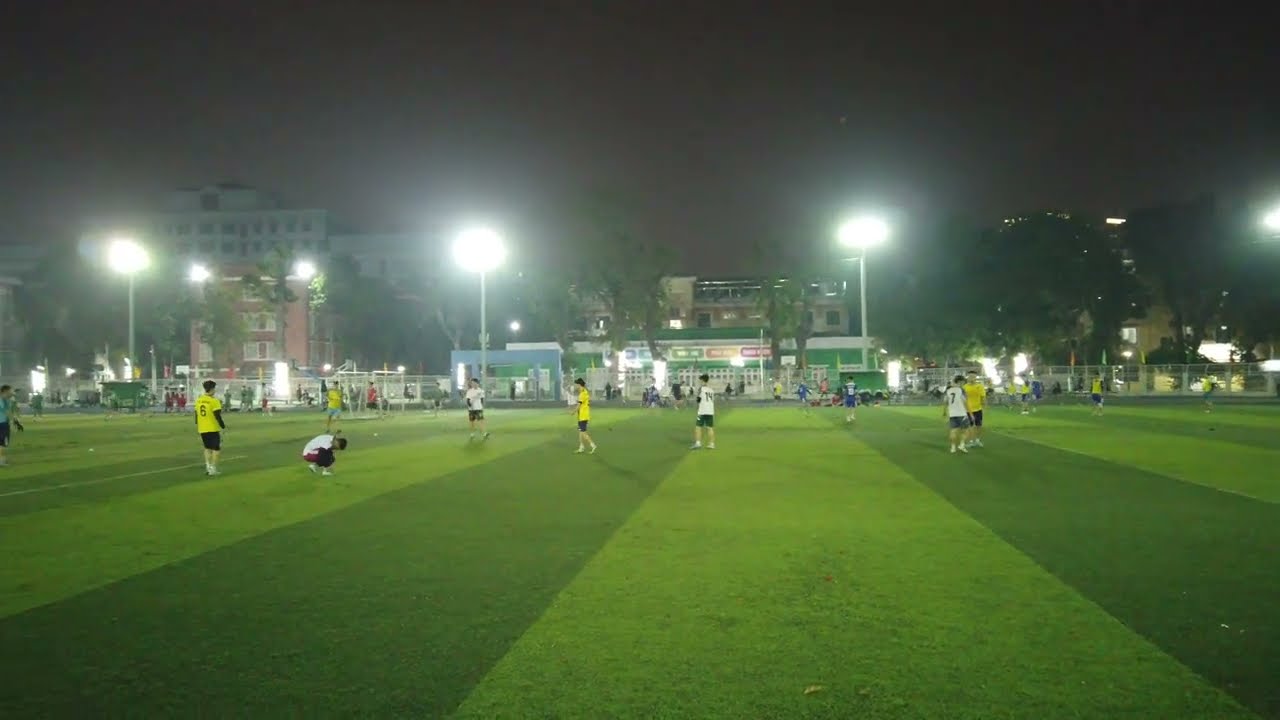This image captures a nighttime soccer match in a well-lit stadium. The field is characterized by alternating vertical stripes of dark and light green grass. Around ten players are visible, divided into two teams: one team is wearing neon yellow jerseys with blue shorts, and the other is in white jerseys with green shorts. The scene is illuminated by several large, glowing white lights, giving a clear view of the action despite the dark and clear night sky. In the background, there are buildings and silhouetted trees, with trees flanking both sides of the field. Behind the players, sparsely attended bleachers are visible, indicating some spectators present. This setup and the outlined details suggest a community field setting, encapsulating the essence of an evening soccer game.